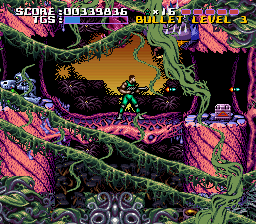This detailed caption could fit the description request:

"A nostalgic screenshot from a classic 2D shooter game, possibly from the late 80s or early 90s, depicting an intense jungle battle scene. The character, clad in a sleeveless green leotard suit, brandishes a formidable machine gun, from which a stream of bullets is actively emerging. He stands poised on a precarious hanging bridge crafted from intertwined red vines, while vibrant green vines crisscross the foreground and drape vertically from the lush canopy above, reinforcing the dense jungle atmosphere. The backdrop reveals a luminous sunset, casting a warm glow across the landscape. Displayed at the top of the screen are essential game metrics including the score, labeled as 'TGS,' the bullet level set at '3,' and a health bar, all providing vital information for the player."